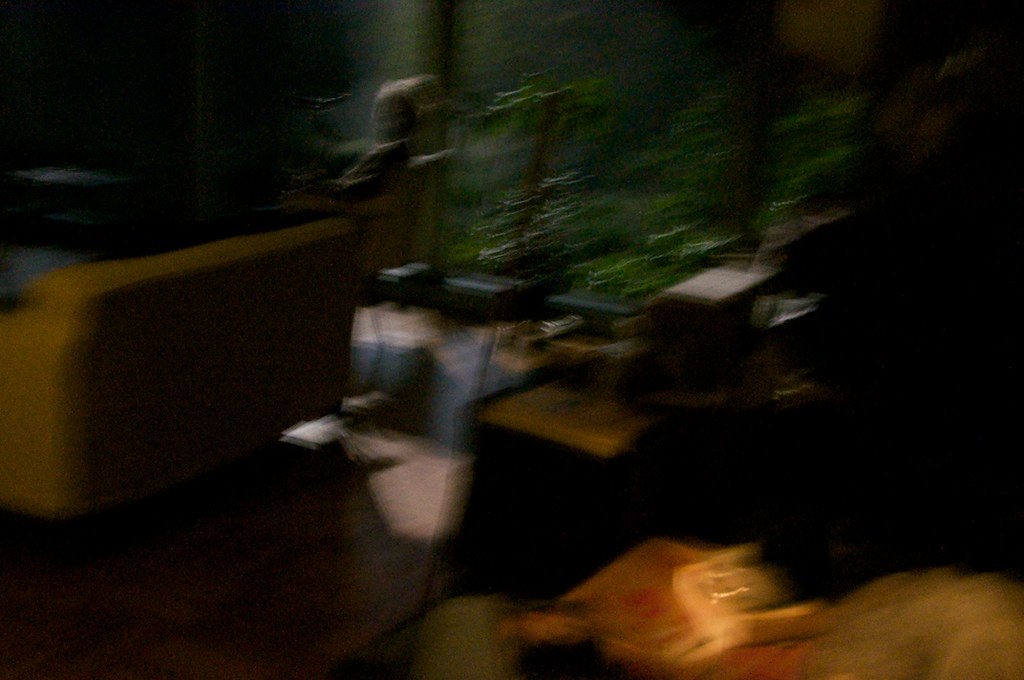An abstract oil painting portrays a contemplative Black man seated in his living room, clad in a sharp black suit. The scene is slightly warped, adding an air of surrealism. He sits thoughtfully in an armchair, illuminated solely by soft moonlight streaming through expansive floor-to-ceiling windows that reveal a dense forest outside. To his left, a pristine white two-seater sofa contrasts against the room’s dark ambiance. A desk to his side is adorned with various miscellaneous items, each gently touched by the ethereal glow of the moonlight, which serves as the only source of illumination on this quiet night.